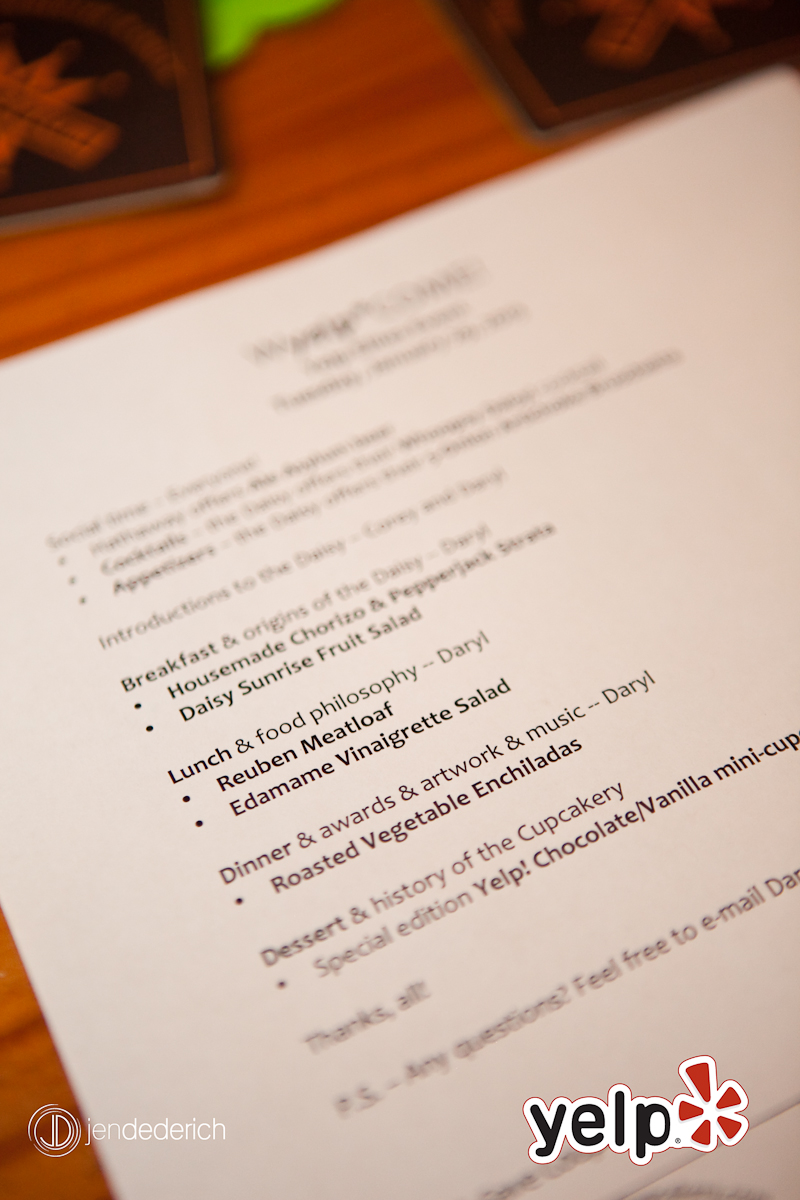The photograph in question is a portrait-oriented color image of a menu, placed on a wood grain tabletop, viewed at a slight angle (approximately a 10:30 or 11 o'clock position). The menu, printed on white paper with black text, is mostly blurry, making it difficult to read in many areas. However, several details are discernible. The visible portions of the menu list various meal options: beginning with "Breakfast" and "Origins of the Dairy," then "Homemade Chorizo and Pepper Jack" and "Daily Sunrise Fruit Salad and Blackcurrant." The menu continues with "Dinner," "Awards," "Artwork," and "Music," followed by "Roasted Vegetable Enchiladas." Under the "Dessert" section, there is a mention of the "History of the Cupcake" and a "Special Edition, Yelp! Chocolate Vanilla Mini," although it cuts off there. The bottom of the menu features an out-of-focus note saying "Thanks All" and "PS-Any Question? Feel free to email." In the bottom right corner, the Yelp logo with its distinctive red flower design is visible next to the word "Yelp," along with an additional logo for Jen Dederich, marked by the text "Jen Dederich" beside a "JD" inside a white circle. The background includes some out-of-focus objects, adding to the composition's everyday realism and atmospheric depth.